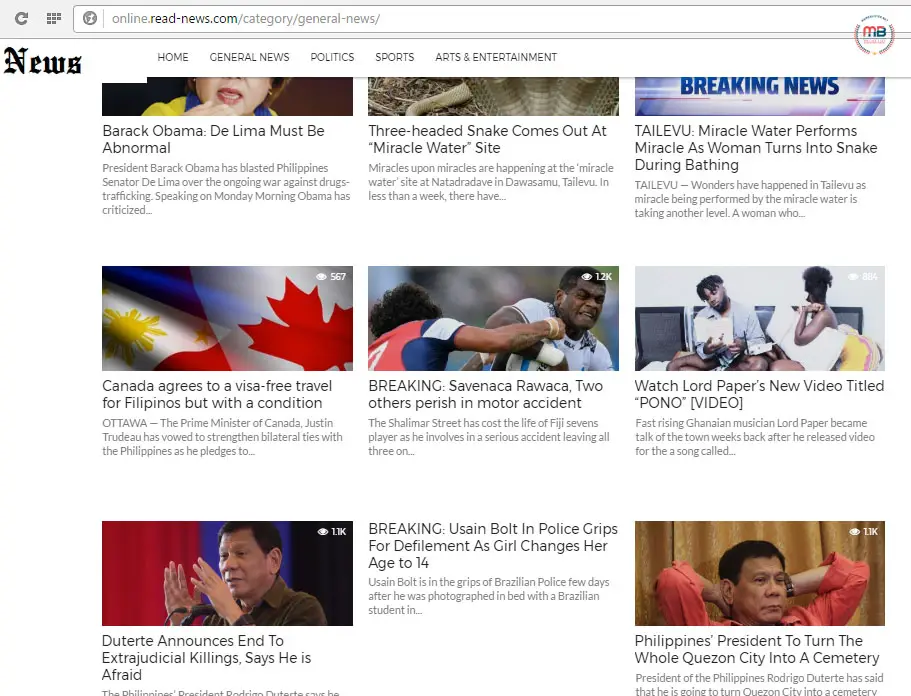This is a cropped screenshot of a news website displayed in a web browser. The browser's search bar indicates the URL as "online.read-news.com/category/general-news/". At the top left corner of the webpage, the word "News" is prominently displayed, while to its right, there are five navigation categories listed in small grey letters: "Home," "General News," "Politics," "Sports," and "Arts and Entertainment." Below this navigation bar, the page shows a series of thumbnails, which include both photos and videos, accompanying various news stories. You can see the bottoms of these thumbnails along with their headlines and brief excerpts, as the page appears to be scrolled down partially, cutting off the full view of the thumbnails. The central part of the screenshot features three prominent news stories, while three additional stories at the bottom are slightly cut off, indicating more content further down the page.